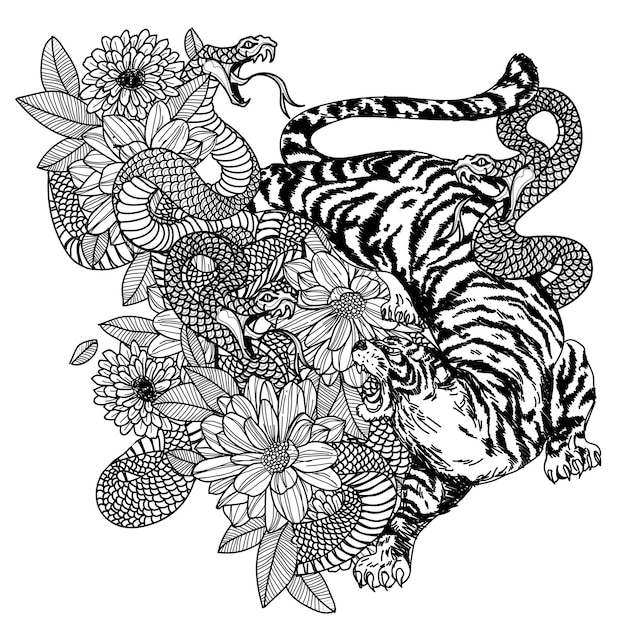This black and white ink illustration, evocative of traditional tattoo or coloring book art, features an intricately detailed scene. On the left side, there is a vibrant array of flowers, resembling zinnias and daisies, interwoven with at least three serpents. One of these snakes is prominent at the top, displaying an open mouth, fangs, and a flickering tongue, while the others coil among the petals and greenery. On the right side, a formidable tiger, characterized by its menacing growl and sharp claws, dominates the scene. The tiger's form curves from the middle top to the bottom, with its tail looping back up to the upper right corner. Notably, another snake coils along the tiger's right side, adding to the dynamic tension in the image. This detailed composition, with its bold lines and intricate patterns, is well-suited for a tattoo or a coloring book.